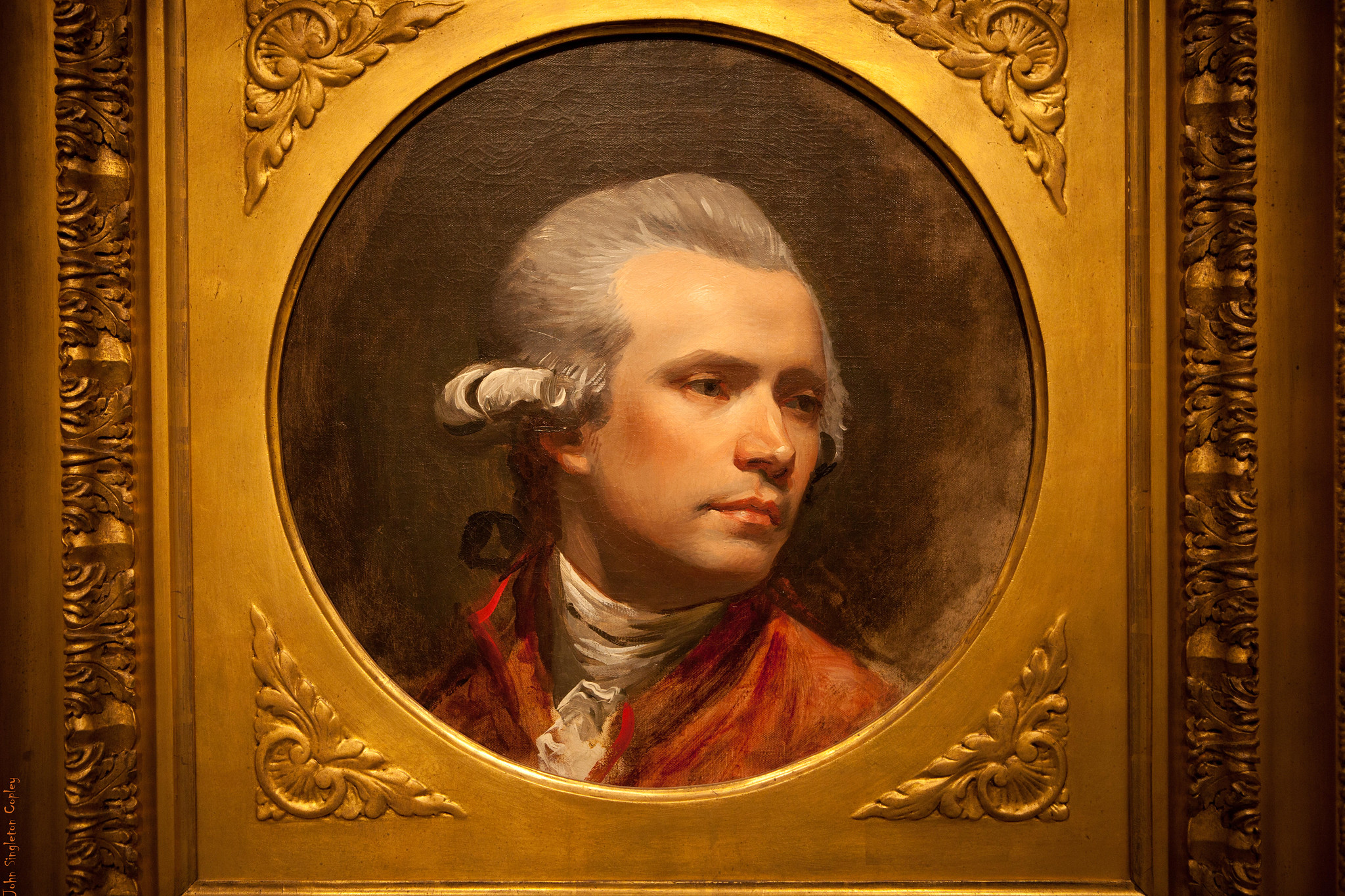The image appears to be an 18th-century vintage painting, likely depicting a notable American or British figure from that era. The central focus is an oval-circular painted portrait of a man with white, curled hair characteristic of the period's style. He is dressed in a red gown over a white outfit, gazing to the right against a grayish-black background. The painting is set in a golden frame with intricate royal designs and patterns, including stylized filigree on both sides. The frame features triangular embellishments at the top and bottom, adding to its ornate and regal appearance. This gold-colored frame gives it a distinguished, historical aura, reflecting the grandeur of the bygone era.